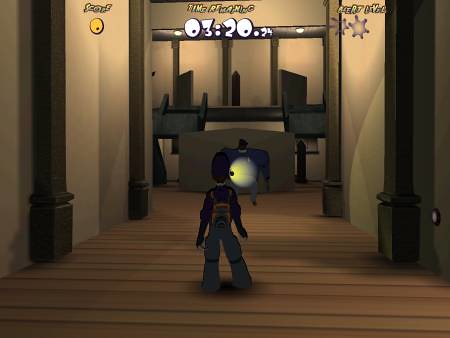This image is a detailed, computer-generated screenshot from a video game, depicting a high-ceilinged interior hallway with wooden walls and floorboards. At the center of the scene is a character seen from a third-person perspective. The character, wearing long jeans, a sweater, and a backpack, stands facing away from the viewer. They seem to be looking towards a much wider, stout, and cartoonish character dressed in dark blue with a hat and gray overalls accented with yellow stripes. This second figure is holding a yellow light or flashlight, illuminating the scene.

The walls of the hallway are a light whitish-brown, and there are dark gray pillars spaced along them. At the top of the image, white text reading "3:20" is prominently displayed, likely indicating the time remaining in the game. In the top left corner, a small yellow circle with a dark dot in the middle appears, along with some indecipherable white text. Additionally, near the top right corner, there are six light purple stars. The score, shown at the top left corner, is zero.